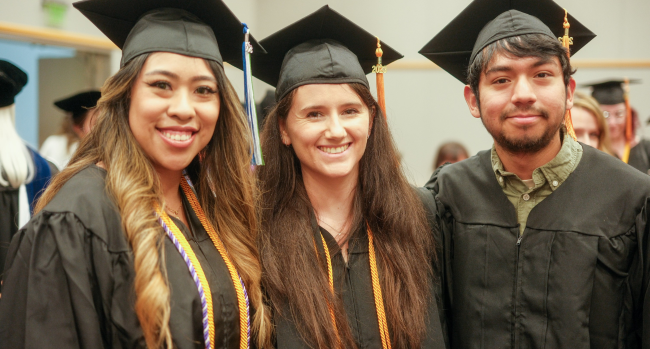This photograph captures a joyful moment of three friends celebrating their graduation indoors, likely a college graduation. All three individuals are dressed in black graduation caps and gowns. The woman on the left appears to be Asian with long brown hair and is wearing makeup. She is smiling broadly, showing her teeth, and she has two honor cords draped around her neck - one purple and white striped and the other gold. The woman in the middle, who is white with long brown hair hanging below her shoulders, also has two gold honor cords. She too is smiling broadly, displaying her teeth, and has a black graduation cap. The man on the right, with brown skin and short dark hair, is also dressed in a black graduation cap and gown. Under his gown, he is wearing a green collared button-down shirt but has no visible cords. He smiles gently, though his teeth are not visible. In the blurred background, other graduates and guests are also celebrating, contributing to an overall atmosphere of happiness and joy.